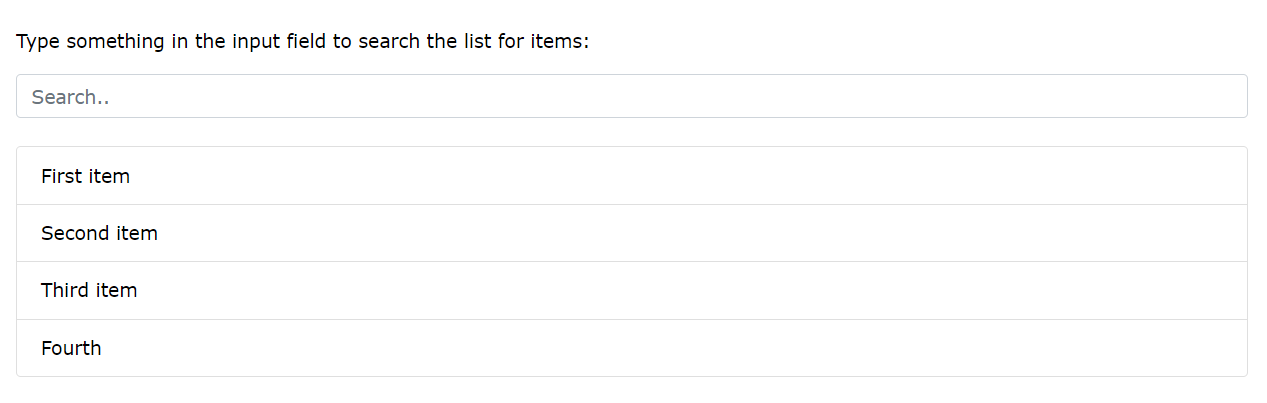The image showcases a minimalistic and simple webpage design. At the very top, there's an instruction reading: "Type something into the input field. Search the list for items." Directly beneath this instruction is a wide search bar with the placeholder text "search" in light gray, inviting user interaction. Below the search bar, no search query has been entered, so a list of placeholder items is visible. These items are labeled "first item," "second item," "third item," and "fourth item," respectively. Each item is encased in a very thin outline, giving them a defined but subtle boundary against the stark white background. The overall color scheme is black font on a white background, emphasizing simplicity and clarity, potentially indicating that this design is a usability test for a website. The spacious layout and broad elements suggest an aim for ease of use and accessibility.